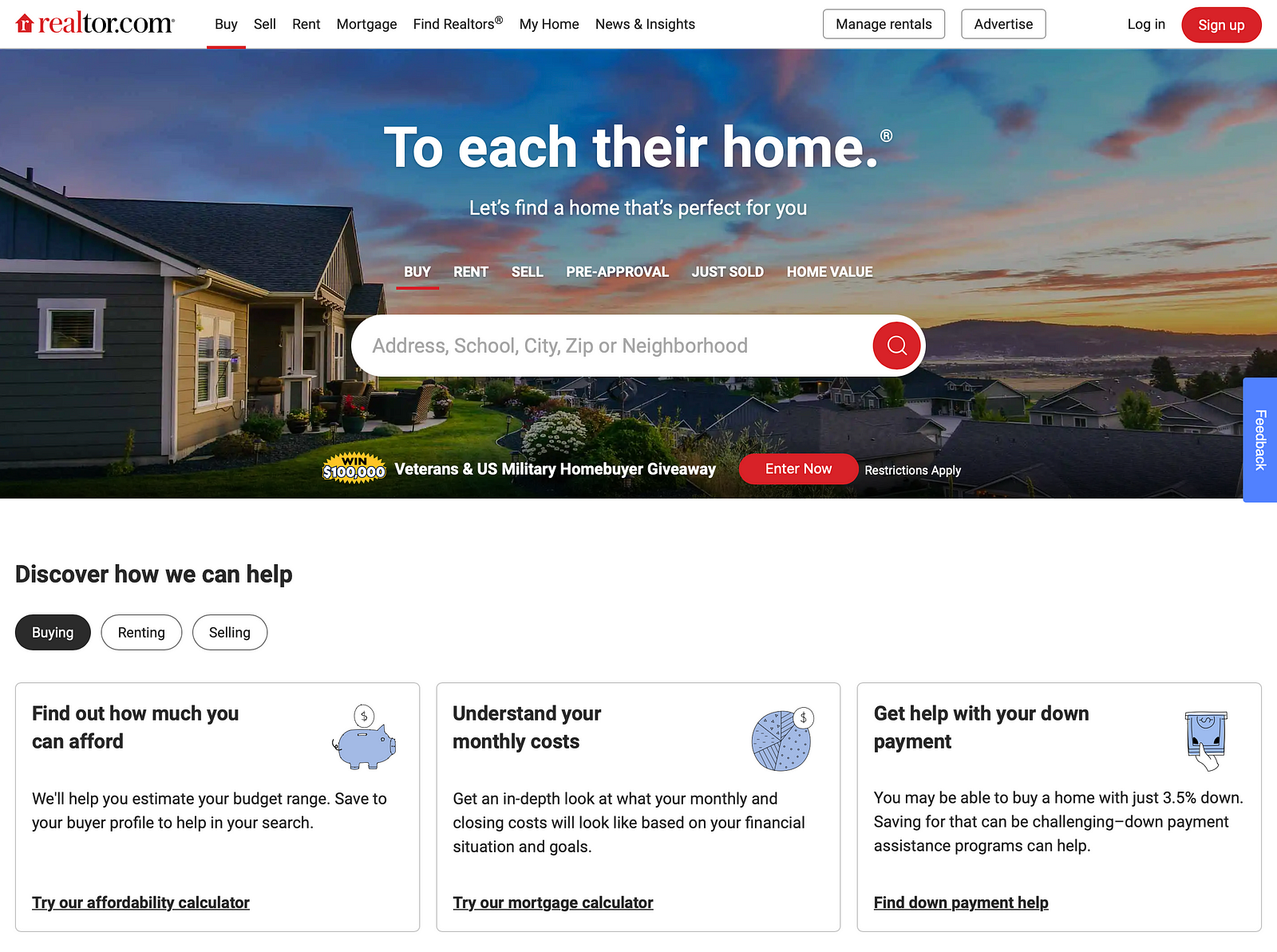Screenshot of Realtor.com Homepage

The Realtor.com logo is prominently displayed in the upper left corner, followed by navigation options labeled BUY (underlined), SELL, RENT, MORTGAGE, FIND REALTORS, MY HOME, and NEWS AND INSIGHTS. 

A large photograph spans the width of the page, capturing an outdoor scene. On the left side, it features a single-story, olive-colored house accompanied by a well-maintained lawn and bushes. Below, a neighborhood with various other houses can be seen.

The headline text over the photo reads: "TO EACH THEIR OWN, LET'S FIND A HOME THAT'S PERFECT FOR YOU." Below this, additional navigation options are listed: BUY (underlined), RENT, SELL, PRE-APPROVAL, JUST SOLD, and HOME VALUE. A search bar is positioned beneath these options, prompting users to search by ADDRESS, SCHOOL, CITY, ZIP, or NEIGHBORHOOD.

Further down the page, the section "DISCOVER HOW WE CAN HELP" is displayed. The BUYING tab is selected by default, alongside RENTING and SELLING tabs. The section provides tips and tools for prospective buyers, such as:

- "FIND OUT HOW MUCH YOU CAN AFFORD": Accompanied by an image of a piggy bank, this tip helps users estimate their budget range, which they can save to their buyer profile.
- "UNDERSTAND YOUR MONTHLY COST": Illustrated with an image of a segmented circle featuring a dollar sign, this tip offers an in-depth look at potential monthly and closing costs based on the user's financial situation and goals.
- "GET HELP WITH YOUR DOWN PAYMENT": Positioned to the right, this tip provides assistance on down payment options for users.

Overall, the screenshot provides a comprehensive overview of the various tools and resources available on Realtor.com to aid users in their home-buying journey.